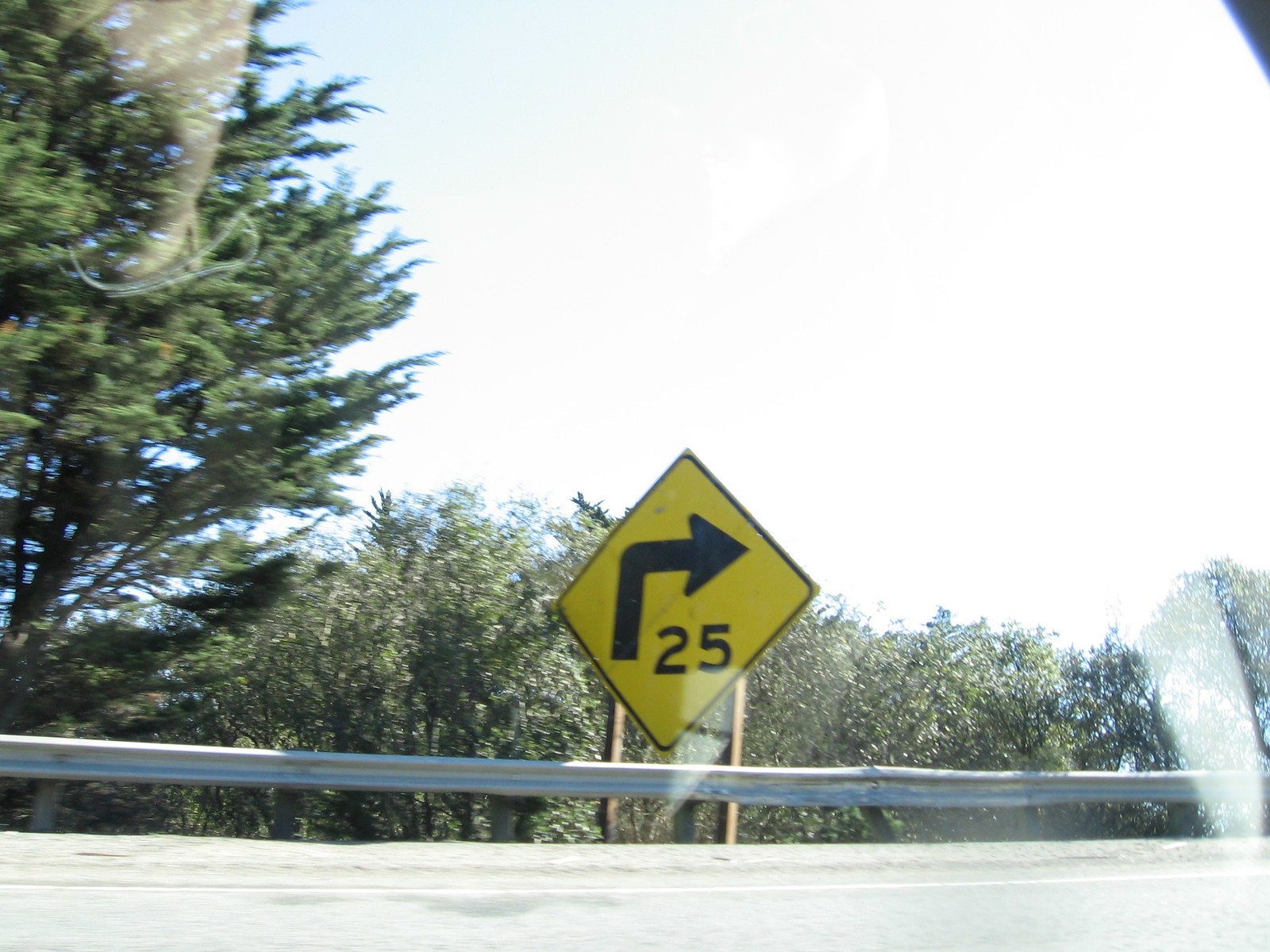This photo, taken from inside a vehicle through a window, depicts a scenic roadside view. In the upper left corner, there's a faint reflection of a person’s arm, clad in long sleeves and a bracelet, against the glass. The reflection is also noticeable in the upper right corner, along with part of the car's interior. 

The left side of the image is dominated by a large green tree, while in the background, numerous smaller trees form a lush green tree line beneath a blue afternoon sky. Prominently displayed towards the bottom is a silver metal road divider, designed to prevent vehicles from veering off the road. Just behind this barrier, which appears slightly elevated, stands a diamond-shaped yellow road sign held up by two metal posts.

The sign features a black arrow that initially goes straight before curving to the right, indicating an upcoming bend in the road. Below the arrow, the sign advises a speed limit of 25 miles per hour to safely navigate the curve. This detailed roadside composition, framed by the car window, captures both the cautionary aspects of the road ahead and the serene natural surroundings.